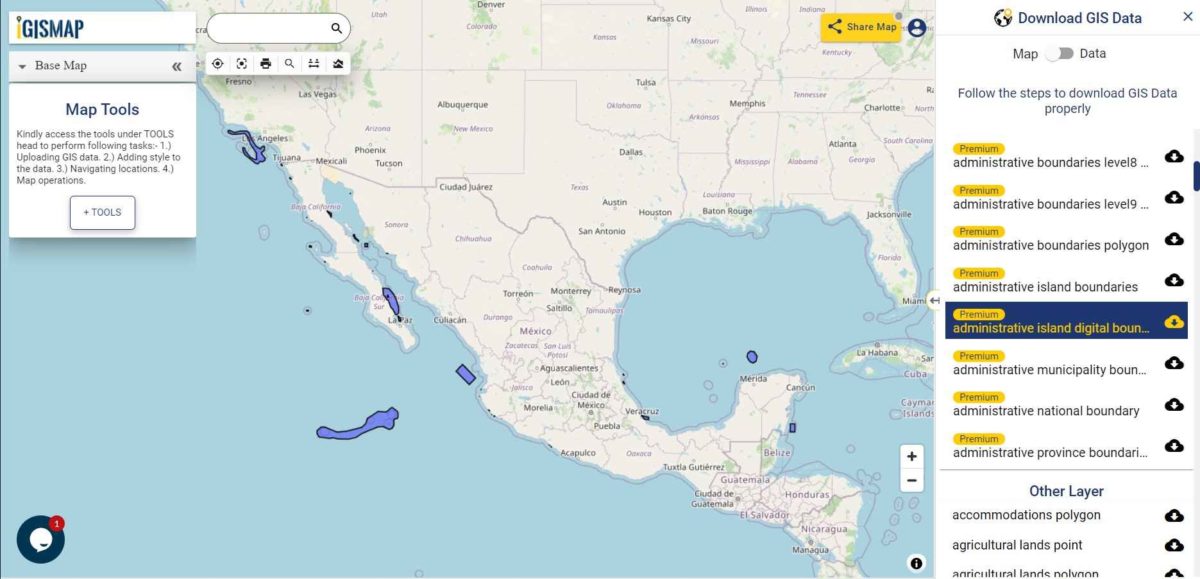**Caption:**

A detailed screenshot from a GIS (Geographic Information System) map interface, primarily focusing on Mexico. The map includes highlighted blue areas in the surrounding waters, indicating specific zones of interest. The interface features several toolbar options along the top and sides, including a base map option, search function, print button, and a share map button located in the upper right-hand corner.

On the right side, a slide-out menu panel labeled "Map Tools" offers various functionalities. These tools enable users to upload GIS data, add styling to the data, navigate locations, and perform map operations. A prominent plus button labeled "Tools" suggests additional functionalities.

Within the slide-out panel, there are multiple vertical options for downloading GIS data, listed under headings like "map" and "data." The interface currently highlights the "map" section, instructing users to follow specific steps for proper data download. Among the listed options, each marked with a premium button, an entry for "Administrative Boundaries Level 8 and 9" is notable. A particular item, titled "Administrative Island Digital Boundaries," is highlighted in blue with yellow text and accompanied by a yellow cloud icon featuring a blue download arrow, indicating its ready availability for download.